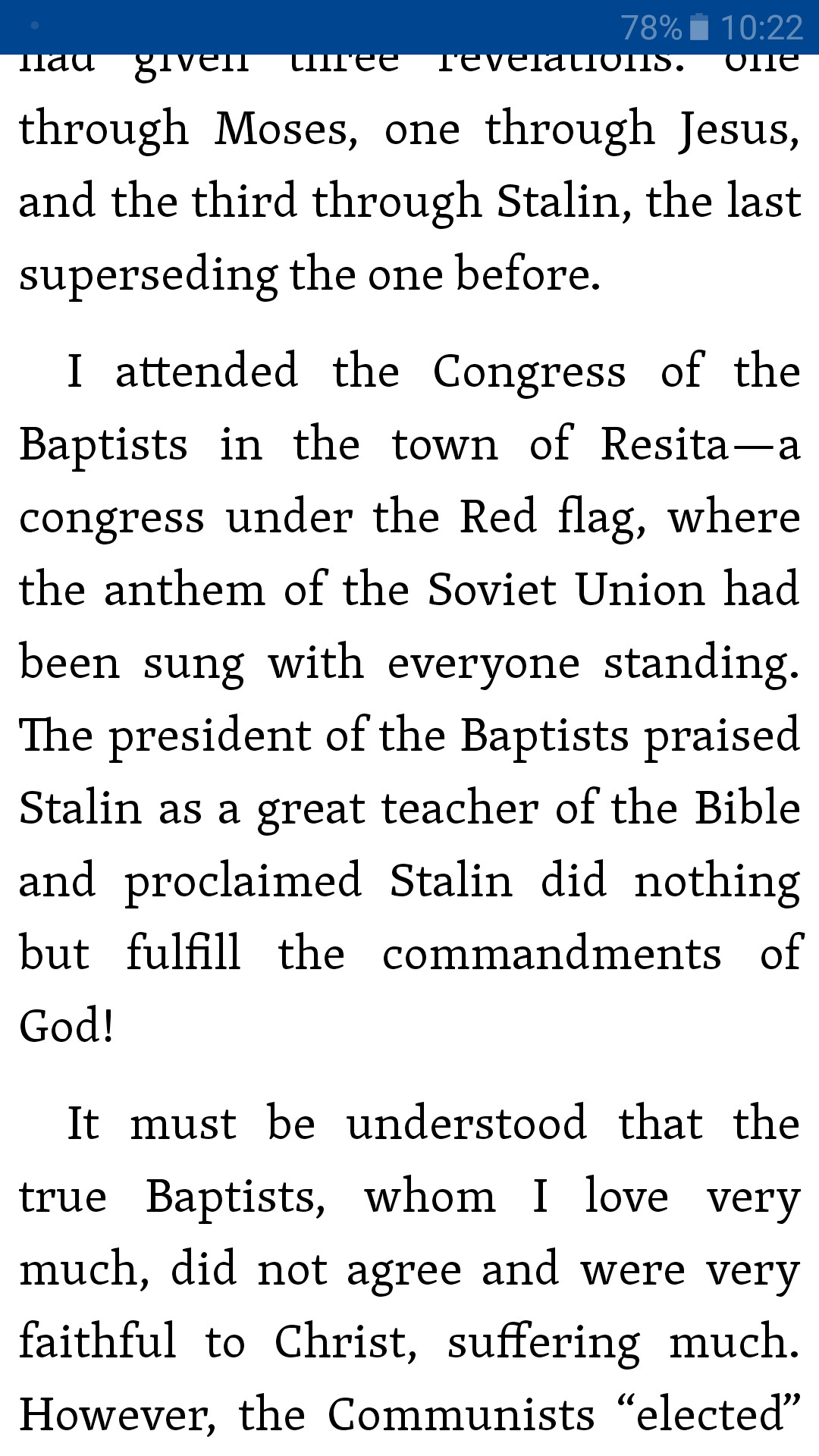This image is a screenshot taken from a mobile phone. Across the top, there's a narrow blue band with lighter blue accents. In the upper right corner, it displays the battery icon indicating 78% charge and the time as 10:22. Below this, the background is white with black text, although the top portion of the text is slightly cut off. The visible text reads:

"through Moses one, through Jesus and the third through Stalin, the last superseding the one before. I attended the Congress of the Baptists in the town of Reseda, a Congress under the red flag where the anthem of the Soviet Union had been sung with everyone standing. The president of the Baptists praised Stalin as a great teacher of the Bible and proclaimed Stalin did nothing but fulfill the commandments of God. It must be understood that the true Baptists, whom I love very much, did not agree and were very faithful to Christ, suffering much; however, the Communists elected."

The detailed description captures the juxtaposition of religious praise and political ideology in the text, highlighting the controversial and historic context of the message.